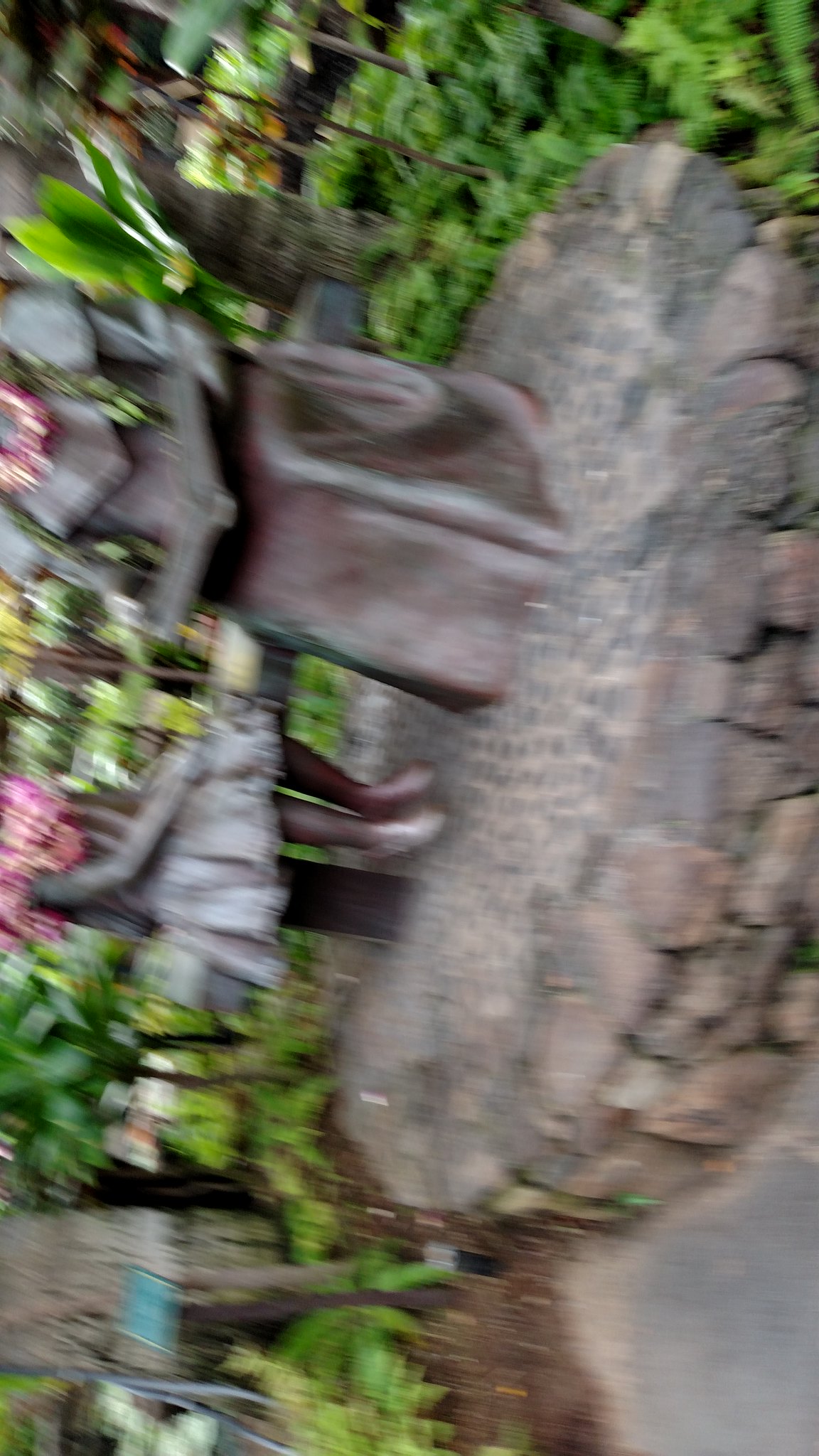This image features an outdoor setting captured at a sideways angle, rendering it somewhat blurry. The central focus seems to be a garden decoration comprising a stone surface on which two carved stone figures are positioned. The details of these figures are vague, but one appears to be an adult, possibly kneeling and clad in a dress, holding an open hardcover book. The head of this figure is not visible. The second figure resembles a little girl, also in a dress, with discernible legs, seemingly seated on a post. Both figures appear to be adorned with traditional floral leis, possibly in shades of purple and white. Behind the stone figures, there's visible greenery and some dirt. Additionally, a short, dark post featuring an informational tag with a green background is seen in the vicinity, although the text on this tag is not legible.